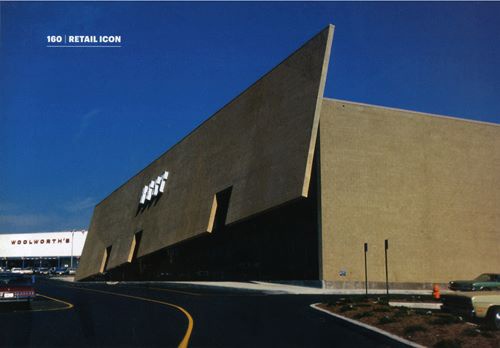This vivid color photograph captures a modern tan retail store on a bright, clear day. The distinct design gives the illusion that the front portion of the building is lifted off the ground, resembling a partially opened garage door with openings for entrances. Prominently displayed on the upper left corner of the building’s facade in white lettering is "160 Retail Icon," underlined with a faint blue line. The store is surrounded by a neatly paved black parking lot lined with yellow markings, accommodating several cars, including tan, blue, and red vehicles. Adjacent to the building on the right is a light gray sidewalk. In the distance, a white building with bold red "Woolworths" signage stands out, surrounded by more parked cars. This arrangement evokes a nostalgic feel, reminiscent of a retail setting from the 1970s.